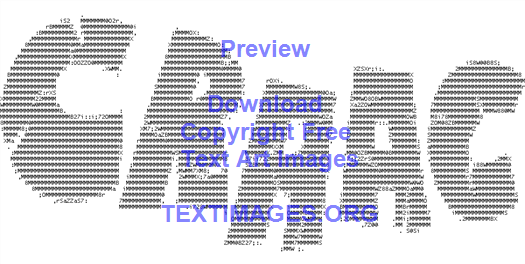The image features an intricate computer-generated design with a white background composed of dots and numbers that, upon closer inspection, spell out the word or acronym "C R A A C" in a wavy form, where the letters seem to dance up and down. The large, all-capital letters "C R A A C" are initially seen in gray-black tones set against a white backdrop. Overlaid on this, in a striking purple-blue font, are the words "PREVIEW, DOWNLOAD, COPYRIGHT FREE TEXT ART IMAGES." At the bottom of the image, in large, bold, all-capital letters, it states "TEXTIMAGES.ORG," indicating the website where users can generate their own text art. This composite preview highlights the functionalities of the website, promoting the creation and downloading of text-based art while emphasizing its copyright-free nature.